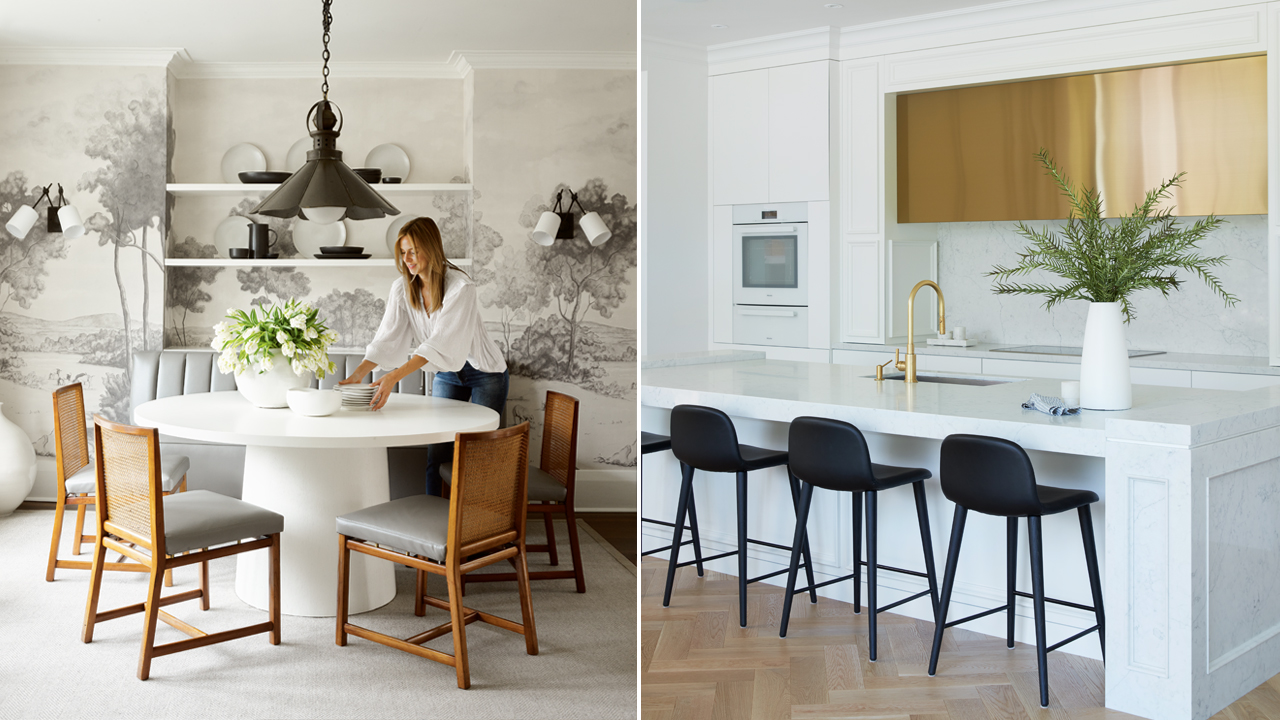The image is divided into two parts. On the left side, there is a modern dining room featuring a round table with a thick cylindrical base, both painted white, though the material is unclear—possibly concrete or wood. Around the table are four brown chairs with mesh backs and dark gray cushions. Behind the table, a gray booth is visible. The table is adorned with a large bowl of white flowers and a few plates being arranged by a lady. The background wall showcases grayish or blackish floral wallpaper, and a built-in cabinet holds black and white plates and serving dishes.

On the right side of the image, a sleek, contemporary kitchen is displayed. The focus is on a white kitchen island complemented by three to four black stools. A white vase with green fern-like plants sits on the island, and nearby is a sink with a golden or copper faucet. The background includes stainless steel appliances, possibly an oven or microwave, contributing to the kitchen's modern aesthetic.